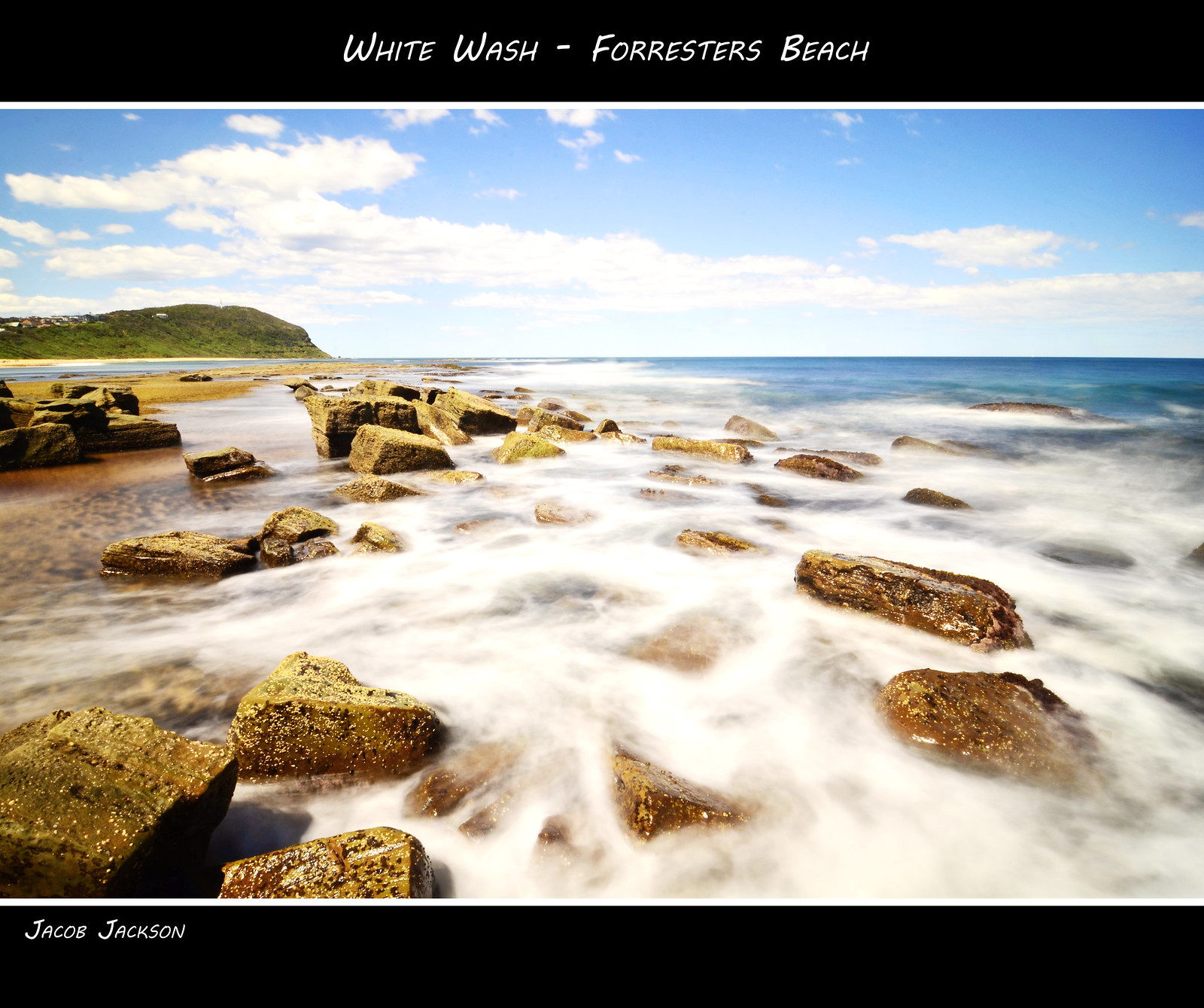The photograph captures a mesmerizing seascape in landscape mode, framed with thick black borders on both the top and bottom. In white text, the top border is labeled "Whitewash – Forester's Beach," while the bottom left of the lower border credits the photographer, Jacob Jackson. The image prominently features an ocean filled with numerous rough, scattered rocks and a milky white froth enveloping the water, giving an impression of fog or smoke on the surface. To the upper left of the image, a green hillside extends into the distance, with a strip of sand at its base, adding a touch of earthy tones to the scene. The sky above is mostly clear with a few white clouds adorning the blue expanse. The water is particularly striking with its transition from the frothy foreground to the clear, deep blue ocean in the distance, creating a natural yet surreal effect.